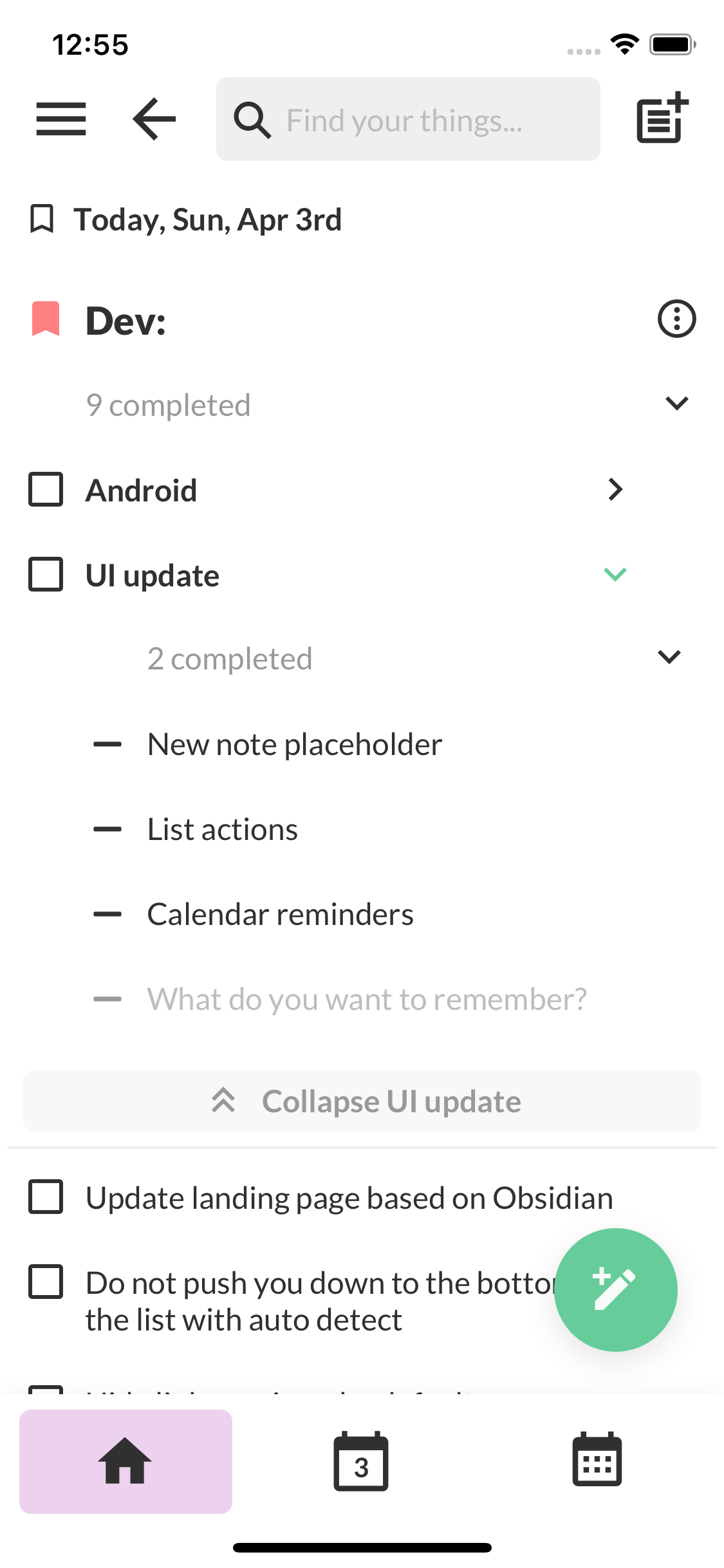The image displays a mobile app interface, presumably a planner or agenda application, aimed at assisting users in managing their tasks and goals. At the top, there is a search bar labeled "Find your things" for locating specific entries. The main part of the screen is dedicated to a list of tasks and reminders for the current day, specified as "today, Sunday, April 3rd."

The app seems to cater to an Android developer, as suggested by some task labels: "Dev," "UI update," and specific project-related tasks. The UI update section expands to show subtasks, including completed tasks like "new note placeholder" and "list actions," while incomplete tasks such as "calendar reminders" are still pending. 

Below the list of tasks, there are additional items like "update landing page based on Obsidian," which users can check off when completed. This interface allows users to track their progress in an organized manner precisely.

At the bottom of the screen, navigation tabs are present including options like "Home," "Calendar," and potentially other categorical views. This navigation provides easy access to different aspects of the user's schedule and tasks.

Overall, the app presents itself as a comprehensive tool for goal tracking and task management, specifically useful for professionals working on detailed projects.